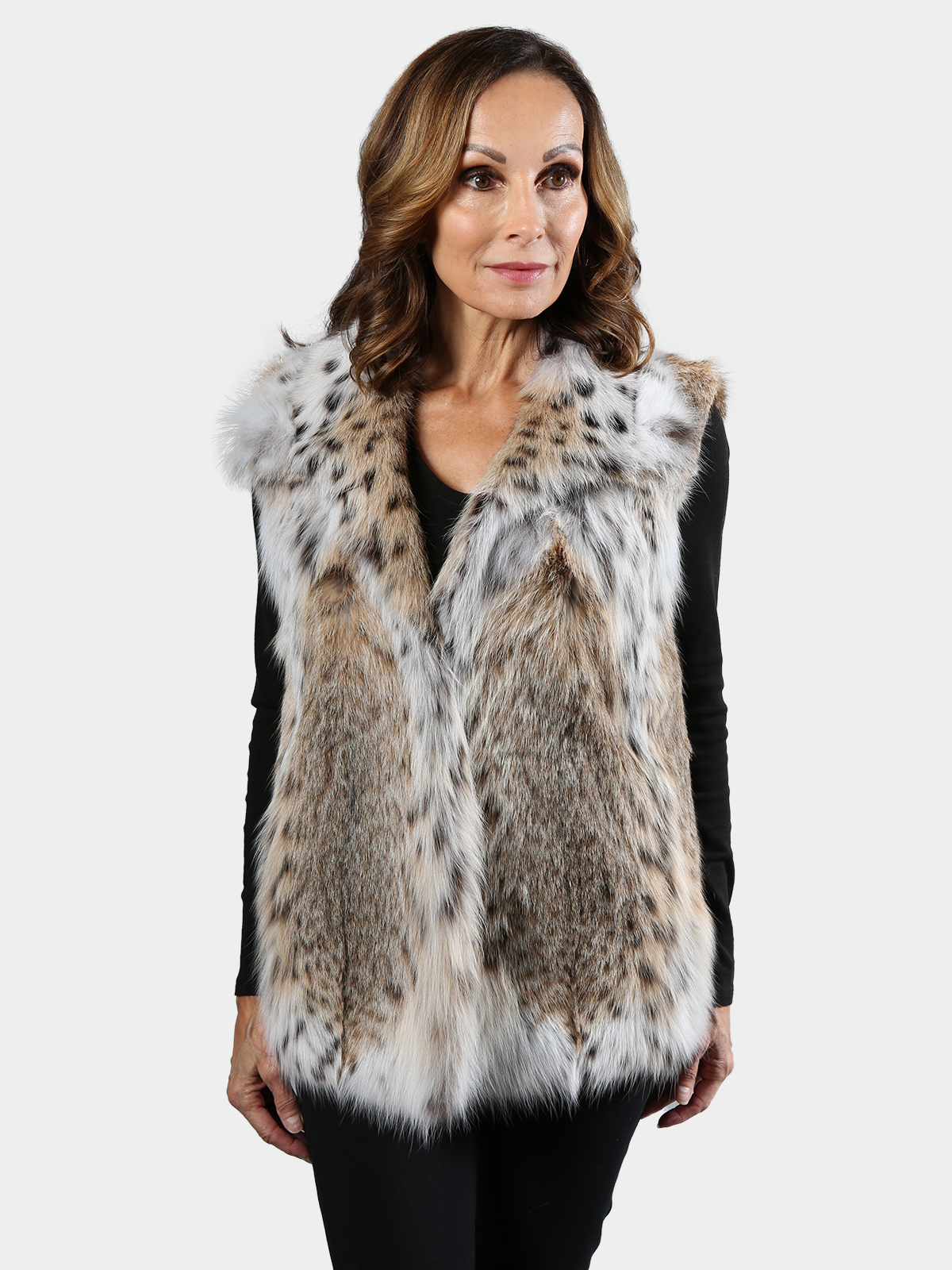The image depicts a middle-aged woman, possibly in her 60s, standing and looking off to the right with a hint of a smile on her face. She has shoulder-length brown hair, curly-ish with very dark, defined, thick eyebrows, and wide-open brown eyes accentuated by makeup, including red lipstick. She's wearing a black long-sleeve shirt and black pants. Draped over her shoulders is a statement piece fur vest extending just below her waist, richly patterned with a mix of white, gray, brown, tan, and flecks of black, resembling animal pelt with spots and stripes. She stands upright with good posture, her hands resting by her sides. The background is a plain off-white, and the vertical image is cropped at her knees. There are no additional elements in the photo, emphasizing the woman and her attire.